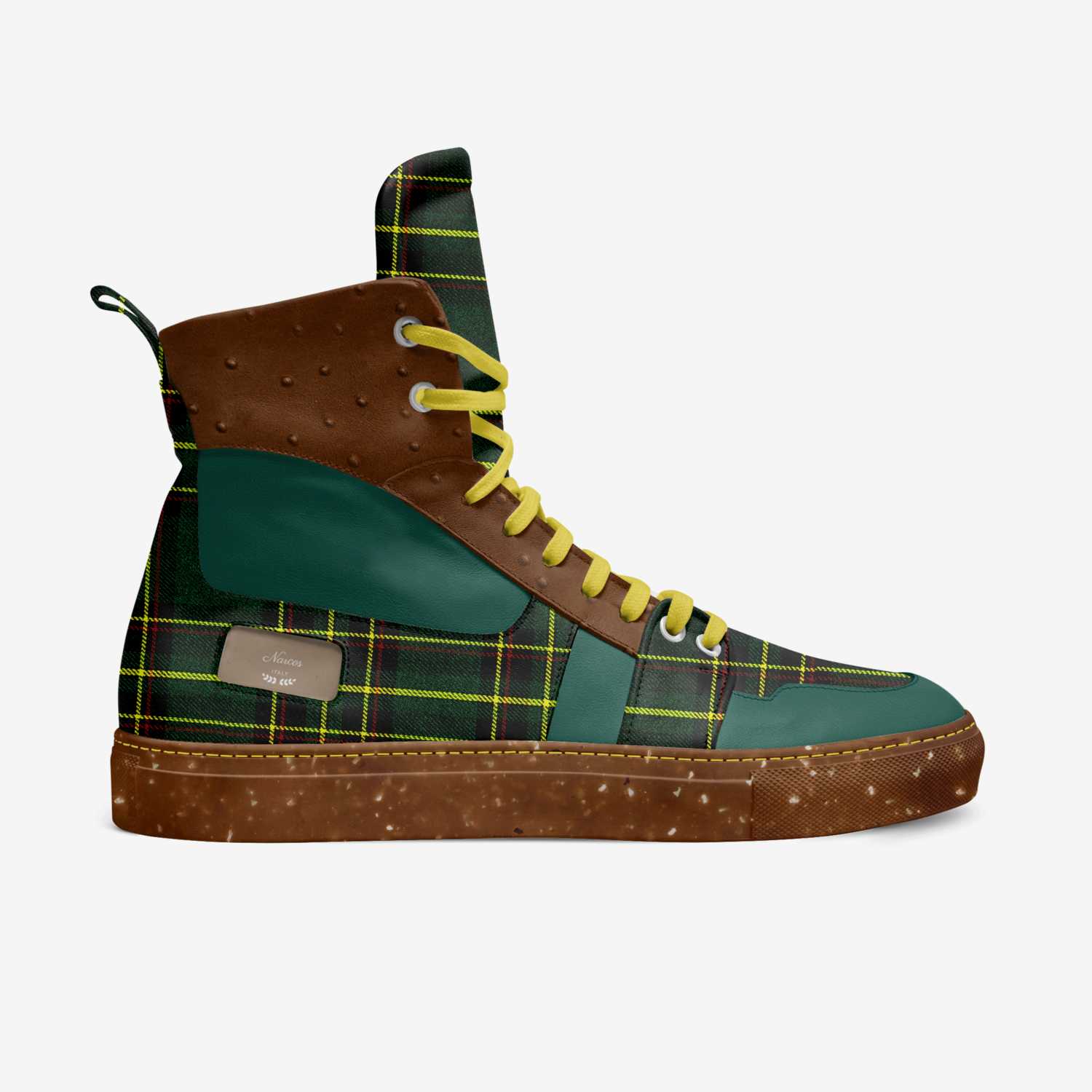The image showcases an up-close, side view of a high-top boot against a light gray background. The boot's design uniquely merges diverse elements, providing a visually captivating display. The sole is predominantly medium brown with scattered white spots, complemented by patches of dark green. Above the sole, the main body of the boot features a vibrant plaid pattern in green, yellow, red, and blue hues, reminiscent of the style of Converse shoes but more robust and less flat. The boot's front section incorporates mixed shades of green and purple, while a strip of blue runs through the middle. Yellow shoelaces weave up to the mouth of the boot, which is adorned with the same plaid pattern. A small gray tag can be seen on the shoe, and atop, the darker brown upper part of the boot encloses a tongue that echoes the plaid design. Despite containing some script or writing, the specifics remain unclear. The overall construction exudes a blend of leather and sturdy material, rendering it not only unique but also stylish.